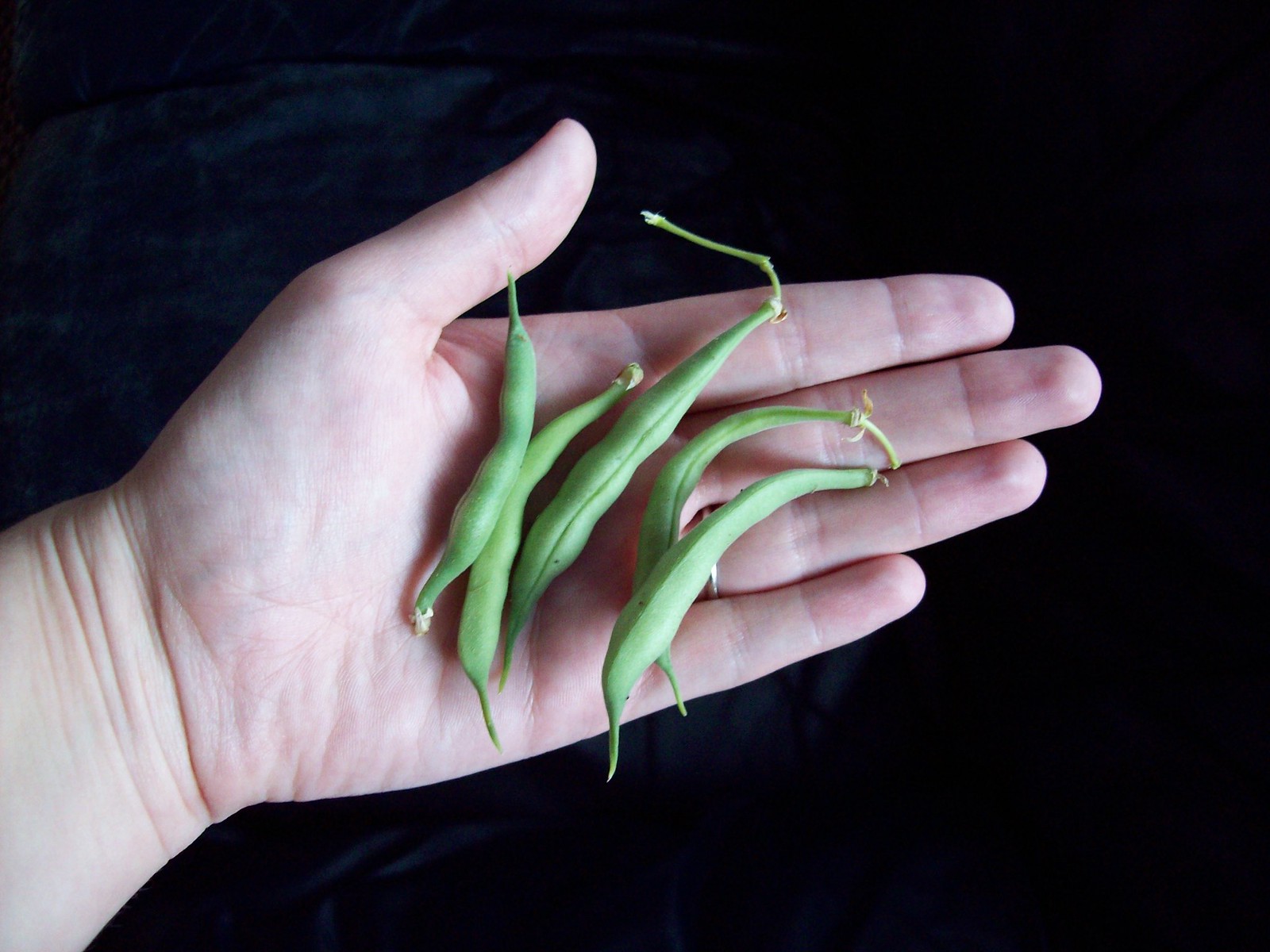A photograph features a woman's left hand, palm up and fingers spread, holding five vibrant green pea pods. These pods, each between two to three inches long, are arranged diagonally from the bottom left to the top right of the image. The pods are slightly bumpy in the middle and still have small stems attached at both ends. The middle pod stands out as the tallest and longest. The woman's hand, suggesting a lighter skin complexion with subtle red hues visible at her fingertips, extends almost horizontally across a nearly black background, which resembles velvet with hints of darker blue fabric and a few wrinkles. Soft light casts over the scene, highlighting the vivid green of the pea pods and the hand.